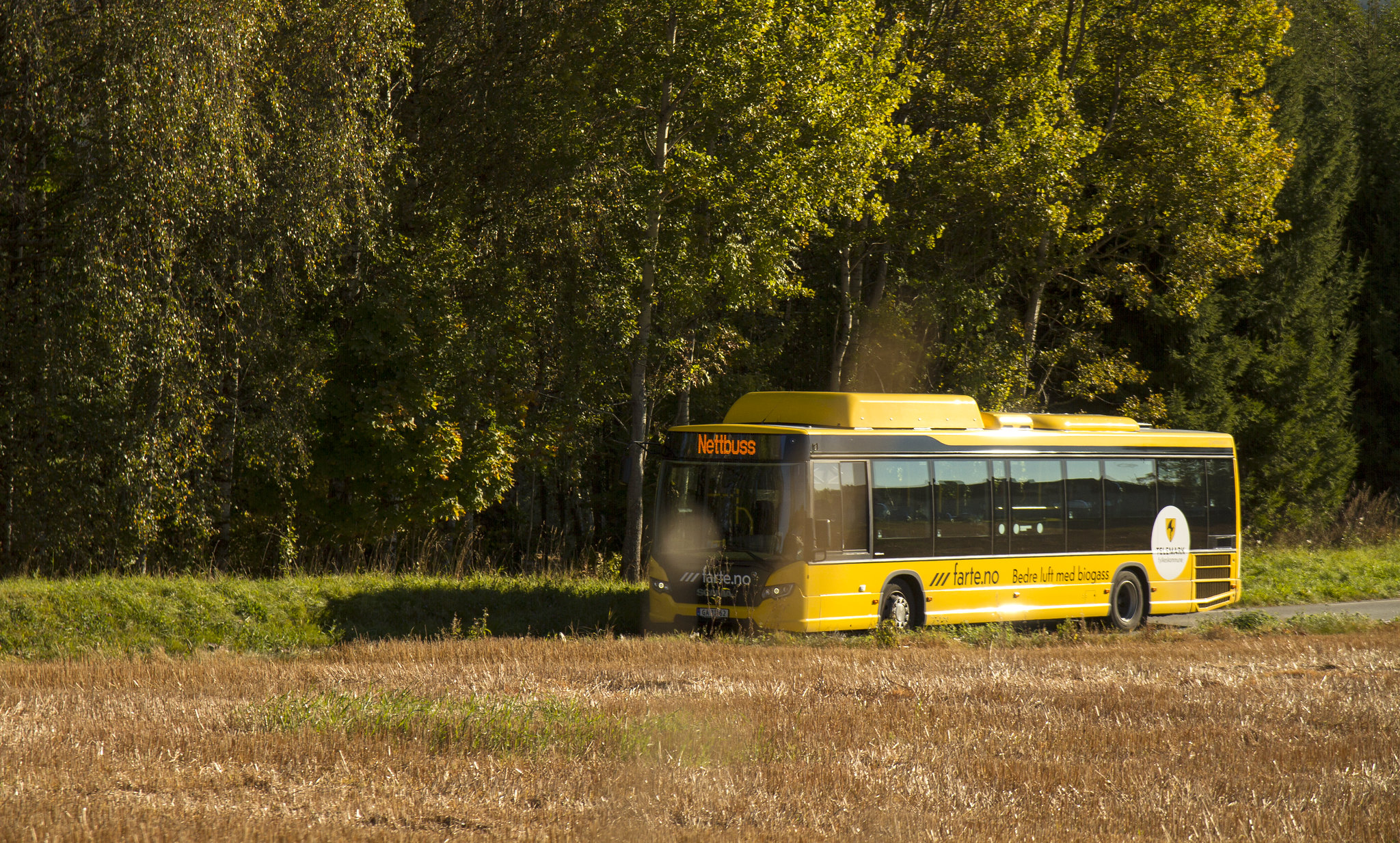The photograph captures a rural scene with a focus on a distinctive yellow bus traveling from right to left. The foreground features a field of predominantly dead, brown grass, with sparse patches of green. Just beyond the field lies a road, upon which the bus is situated. The bus is primarily yellow, with a section of clear glass windows spanning its length for passenger visibility. The lower part of the bus is yellow with two black tires, while the upper portion includes text and possibly storage compartments. Notably, there's a scrolling text display above the driver that reads "middle bus" and another side text, "Fierte.no". Additionally, a white circular logo is visible near the rear right side. Behind the road and bus, a lush green berm rises, leading to a dense wall of tall trees that extend across the background, completing the picturesque outdoor setting.